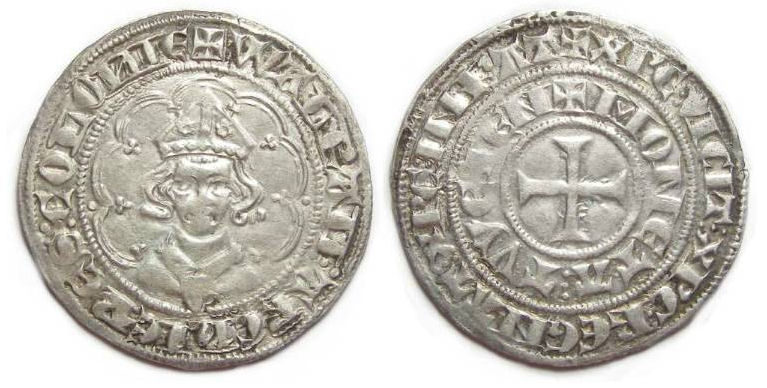This image showcases two silver coins, slightly worn with age, displayed on a white background. Both coins are approximately the size of a half-dollar or dollar coin. The left coin features an etched face at its center, crowned and framed by long hair that reaches the chin, with letters forming a partial border around the top. The coin has a slightly worn right edge with dark markings scattered across its surface. The right coin depicts a central cross on a silver base, encircled by lettering and diverse geometric shapes or symbols etched around the edge. The edges of both coins appear aged and bent, with indents around their centers displaying a darker silver hue compared to the raised areas. Despite their age and the darkened silver, the intricate designs remain discernible yet challenging to fully decode.